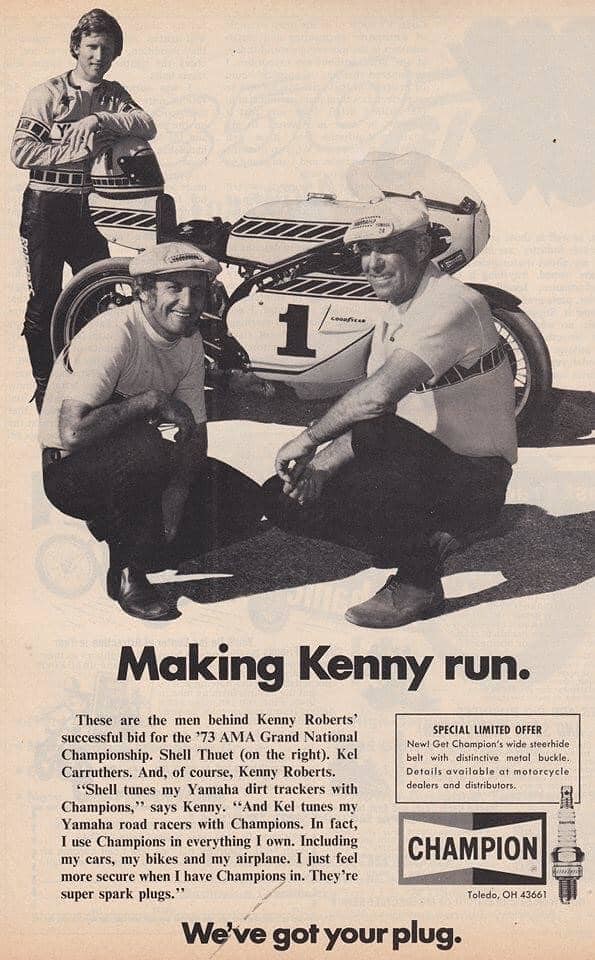The image is an old, black-and-white advertisement that looks like a page from a vintage magazine or poster. It features a motorcycle racing team associated with the 1973 AMA Grand National Championship. The centerpiece is a white race bike with the number one emblazoned on it. Three men surround the motorcycle: two are kneeling in light-colored shirts and dark pants, while the third man, possibly Kenny Roberts, stands in the background leaning against a helmet. He wears a light-colored jacket with square bands around the arm and waist and dark pants. 

The large headline at the top reads, "Making Kenny Run." Underneath, a caption provides context: "These are the men behind Kenny Roberts' successful bid for the '73 AMA Grand National Championship - Shell Thewitt on the right, Cal Carothers, and of course, Kenny Roberts." A direct quote from Kenny Roberts follows: "Shell tunes my Yamaha dirt trackers with Champions, and Cal tunes my Yamaha road racers with Champions. In fact, I use Champions in everything I own, including my cars, my bikes, and my airplane. I just feel more secure when I have Champions in. They’re super spark plugs."

At the bottom right, the advert features the Champion logo and an image of a spark plug, accompanied by the slogan, "We've got your plug." The overall color scheme is a mix of tan, black, gray, and white, contributing to its vintage look.